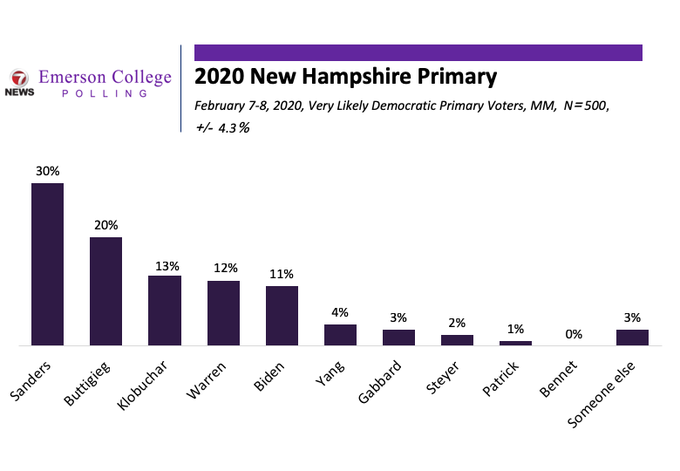This image displays a detailed bar chart representing the political polling results of the 2020 New Hampshire Democratic Primary, conducted by Emerson College and 7 News on February 7-8, 2020. The background is predominantly white, highlighting the information effectively. In the top left corner, the image features the 7 News logo adjacent to purple text reading "Emerson College Polling." To the right spans a purple bar, with black text beneath it detailing the poll specifics: "2020 New Hampshire Primary, February 7-8, 2020, very likely Democratic primary voters, n=500, ±4.3%."

The lower portion of the image contains multiple vertical bars, each accompanied by a candidate's name below and a corresponding percentage above, reflecting their support among the polled voters. The bars, colored in dark purplish hues, vary in height, correlating with their percentage figures. Bernie Sanders leads with a tall bar at 30%, followed by Pete Buttigieg at 20%, Amy Klobuchar at 13%, Elizabeth Warren at 12%, Joe Biden at 11%, Andrew Yang at 4%, and Tulsi Gabbard at 3%. Further down, Tom Steyer stands at 2%, Deval Patrick at 1%, and Michael Bennet at 0%. There is also a category for "Other," collectively accounting for 3%.

This chart visually represents the comparative standing of each candidate in the poll, providing a clear, concise overview of the 2020 New Hampshire Democratic Primary electorate's preferences at that time.